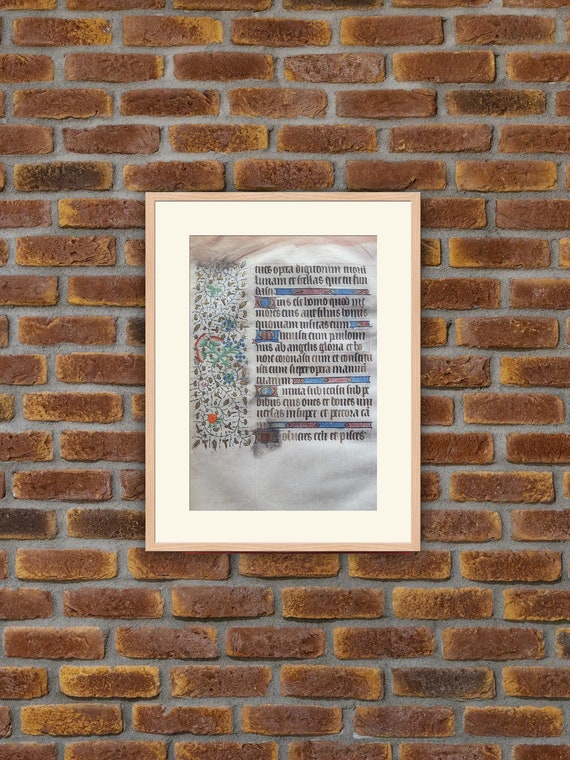This image depicts a red brick wall with thick mortar joints and some yellow highlights on several bricks. Mounted at the center of the wall is a digitally-rendered framed picture, encased in a light wood, tan-colored frame with a white matting. The artwork within the frame features an antique-looking design with unreadable text, possibly in Latin or an old-world style font, set against a cream background. The text is rendered in a brown-black color, appearing somewhat wrinkled as if the paper had been wet. On the left side of the text is an abstract stripe composed of floral and other organic shapes in green, orange, blue, and brown hues. These design elements add a vibrant contrast to the otherwise sepia-toned script and the rustic backdrop of the brick wall, creating a striking visual intricacy.